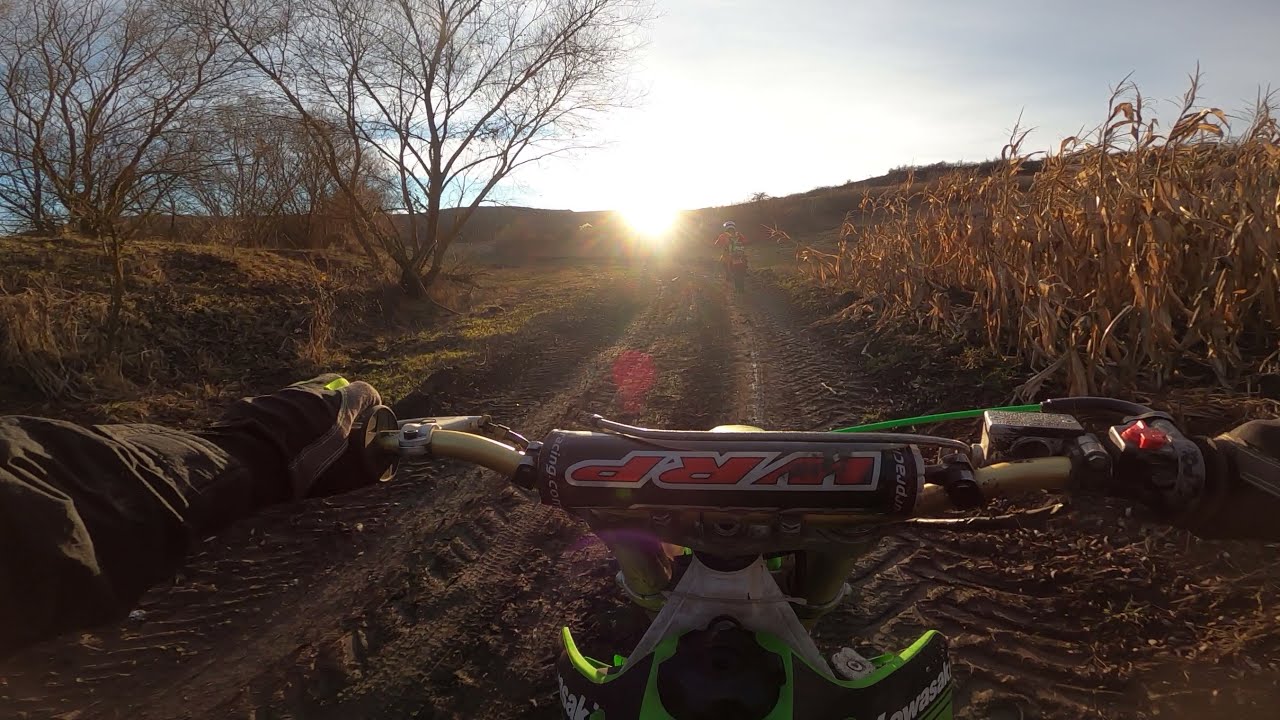The image captures the perspective of a motocross rider looking over the handlebars of their bike, which prominently features the initials "WRP" in red text with a white border. The bike itself is outfitted in black, lime green, and red colors, with notable components in a neon green shade. The rider, wearing black sleeves and black gloves with gray and lime green accents, is navigating a dirt trail marked by large tractor tire tracks. A small camera is attached to the bike's right handlebar. Ahead, another rider dressed in orange with a white helmet rounds a bend. On either side of the trail, detailed scenery includes a grassy field with trees to the left and a cornfield ripe for harvest to the right. The sun graces the horizon, suggesting either dawn or dusk, casting a warm light across the landscape. The sky is bright, adding to the vividness of this outdoor adventure scene.